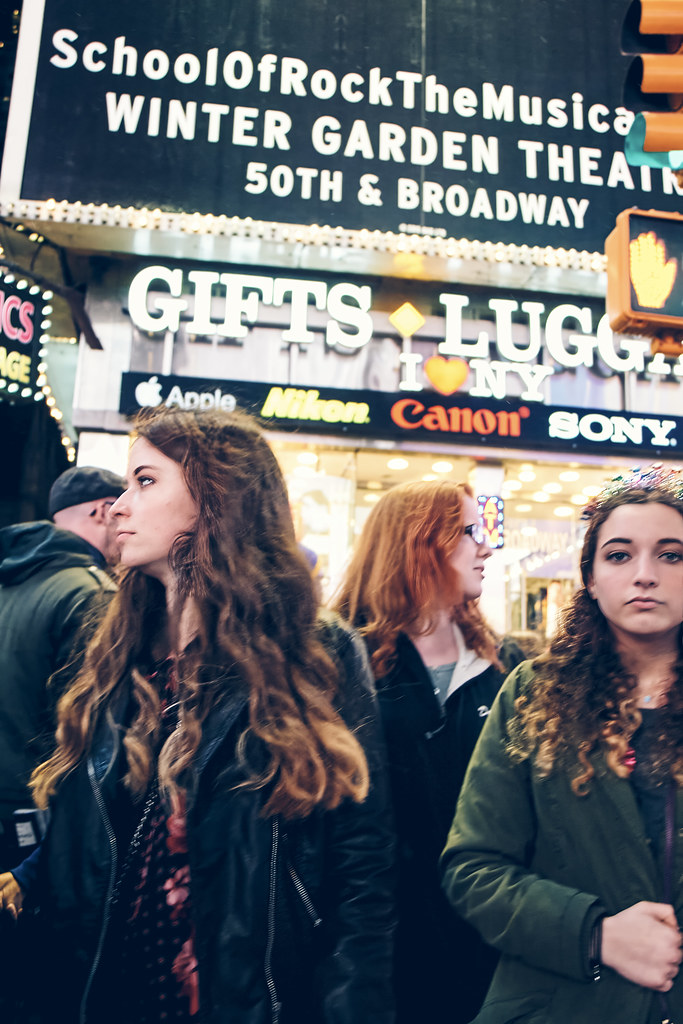This image captures a casual group scene featuring three young women, seemingly in their twenties, standing in front of a large building adorned with bright, eye-catching signage. The setting suggests a busy, urban environment, likely in New York, given the visible signs.

On the left side of the image stands a woman wearing a blue jacket with brown hair flowing over her shoulders. Her body is angled towards the camera, while her gaze shifts to her right, aligning her head in a three-quarters view. 

In the middle, there's a woman with red hair sporting glasses and a dark jacket with a white collar. She is looking off to her right, appearing somewhat preoccupied.

On the right side, another woman faces the camera directly, wearing a green jacket. She has curly brown hair cascading over her right shoulder and clasps her right hand in front of her. Her expression is neutral, suggesting she is caught off-guard by the picture.

In the upper background, a man partially visible to the left is wearing a hoodie and cap, looking towards the camera. Above the group, a prominent black sign with white text reads "School of Rock, the Musical" followed by another sign for the "Winter Garden Theater" at "50th and Broadway". Below, another sign reads "Gifts Luggage", along with company logos including Apple, Nikon, Canon, and Sony. There is also an "I love New York" logo featuring an orange heart. The bright lights and bustling atmosphere reinforce the urban setting of this candid photograph.